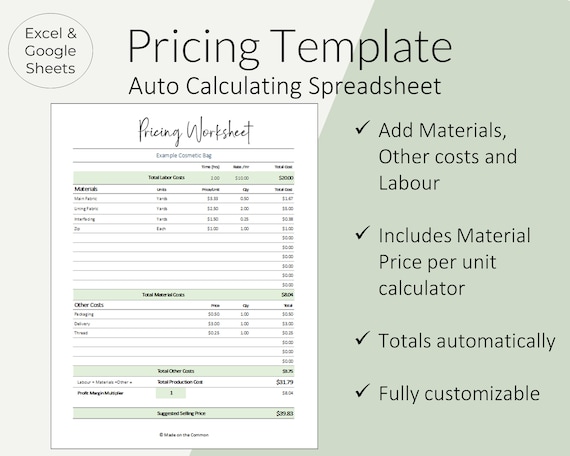This image showcases a detailed pricing template designed for Excel and Google Sheets. The document is split into two background colors: the left side is off-white, and the right side is gray. The top left corner features a black circle with an off-white interior that highlights "Excel and Google Sheets." Across the top, in prominent black lettering, it reads: "Pricing Template Auto-Calculating Spreadsheet."

On the right side of the document, four key attributes are listed next to check marks: 
1. Add Materials, Other Costs, and Labor 
2. Includes Material Price per Unit Calculator 
3. Totals Automatically 
4. Fully Customizable

The left side displays a demo of the actual spreadsheet, titled "Pricing Worksheet." Although the column headings are not readable due to their small size, the form includes fields such as Total Labor Cost, Total Material Goods, Selling Price, and Suggested Selling Price, indicating it’s a comprehensive tool for cost calculation. The overall color scheme consists of light green and light gray hues, with key sections in bold to differentiate the various components of the spreadsheet.